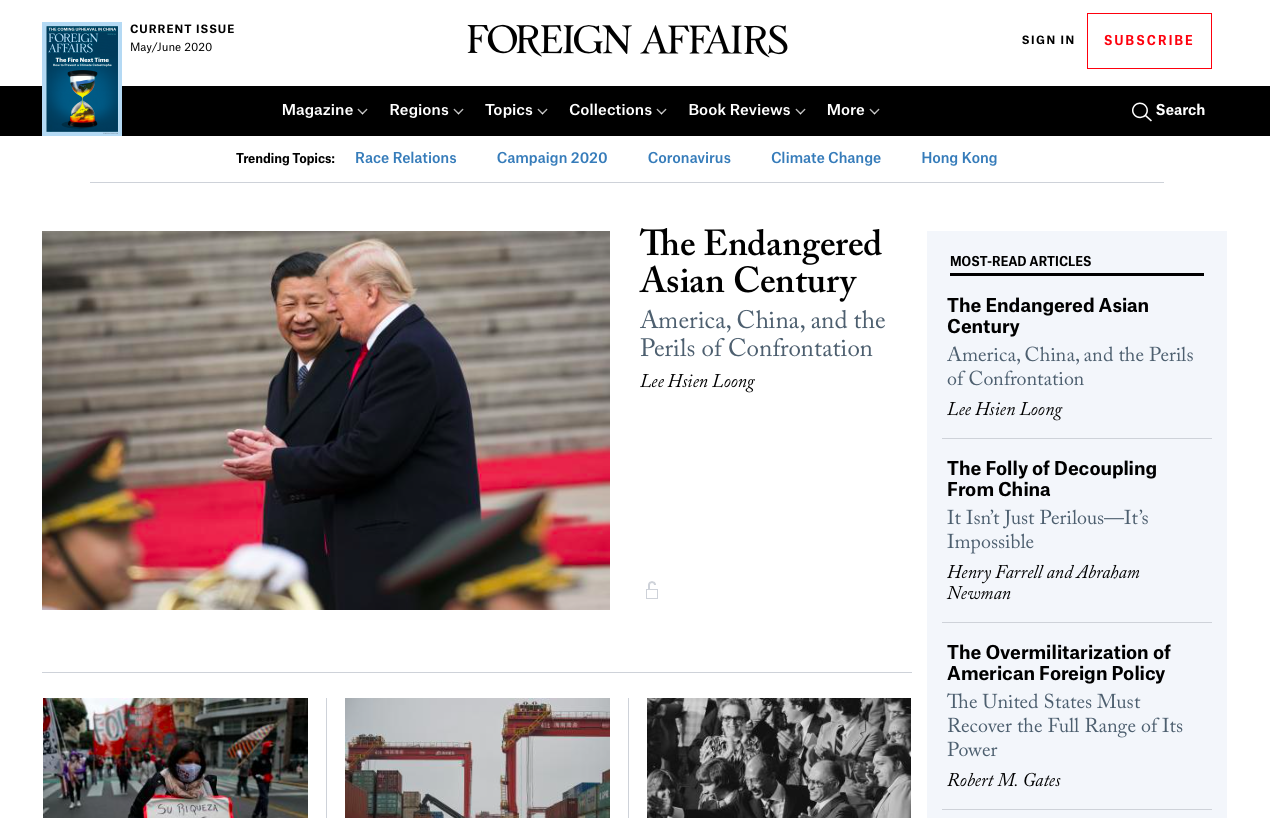This is a detailed caption for the described image:

---

A comprehensive screenshot of the Foreign Affairs magazine webpage is displayed. In the upper left-hand corner, there is a thumbnail image of the magazine cover. The heading reads: "Current Issue: May/June 2020." Below is a navigation bar, with categories labeled: Magazine, Regions, Topics, Collections, Book Reviews, and More.

The main section prominently features a compelling image of Donald Trump alongside the Chinese President, set against a background that underscores geopolitical tension. The bold headline beneath the image reads: "The Endangered Asian Century: America, China, and the Perils of Confrontation."

On the right-hand side of the webpage, there is a vertical list titled "Most Read Articles," which includes the following entries:
1. The Endangered Asian Century
2. The Folly of Decoupling From China
3. The Over-Militarization of American Foreign Policy

Below the main image, three smaller photos are displayed side by side; however, no descriptions accompany these images.

---